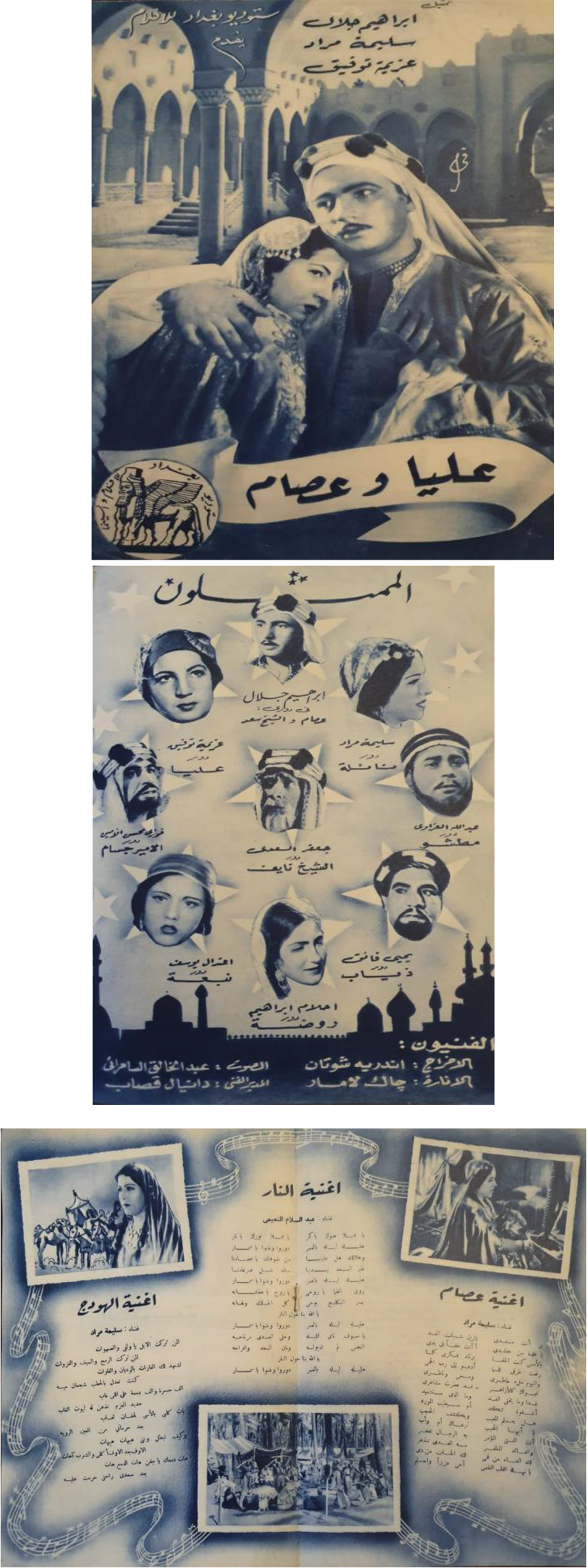The image showcases three sepia-toned illustrations, each approximately two inches wide and three inches tall, stacked vertically. They appear to be vintage promotional materials, possibly for a movie from the 1930s or 1940s, featuring black-and-blue text and imagery on a tan background, with extensive Arabic script.

The top illustration, in black and white, depicts a somber scene with a man in a mustache and sheik's headdress, holding a woman wearing an ornate headpiece and long robes. They are set against an Egyptian-style architectural backdrop of stairs and columns, adding an air of ancient mystique.

The middle poster displays a circular arrangement of disembodied heads—totaling ten, centered around an older man wearing a hat—likely representing the movie's stars. Each head is placed on a star, with Arabic writing under each, possibly identifying the actors. A city silhouette faintly graces the bottom of this piece.

The bottom image, predominantly textual, features a clutter of Arabic script alongside three small inset photographs or drawings, potentially scenes from the film. Music notes encircle the border, adding a decorative touch to the overall design.